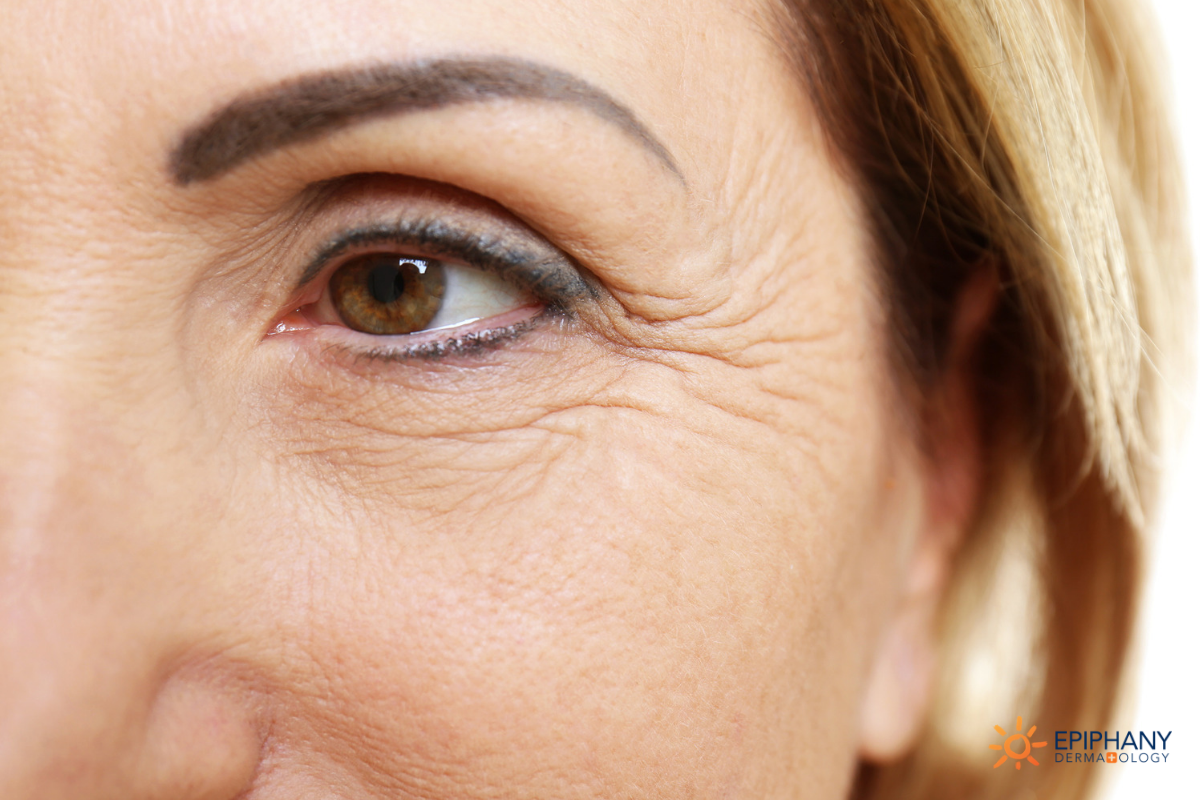This close-up image captures the left eye of an elderly Caucasian woman with fair skin and visible wrinkles, particularly crow's feet extending from the outer corner of her eye. She has light brown eyes, a dark brown eyebrow, and blonde hair. The woman is wearing eyeliner on both her top and bottom lash lines. Only the left side of her face is visible, from her nose to her cheek, and her ear is shown. In the bottom right corner, the image features an orange sun icon with the text "Epiphany Dermatology," suggesting a focus on skincare improvements.